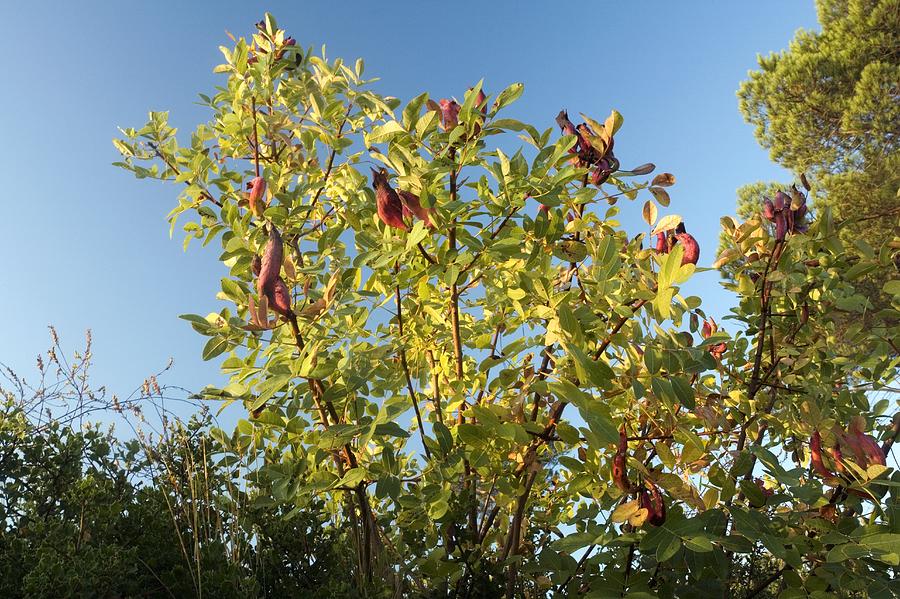This outdoor photograph captures a golden afternoon light illuminating a clear, cloudless blue sky. Taken from a ground-up perspective, the image is centered around a narrow, green tree with thin brown branches and a mix of light green, yellowish, and red leaves. Notably, within this tree are striking maroon and pink flowers that resemble birds in their elongated, sharp-tipped shapes. To the right side of the frame stands a tall green pine tree, its foliage bathed in sunlight. At the bottom left corner of the photograph, a green bush with stick-like structures topped with vivid pink flowers adds texture to the scene. Background shrubbery gives depth, creating a harmonious blend of colors and shapes in this natural setting.